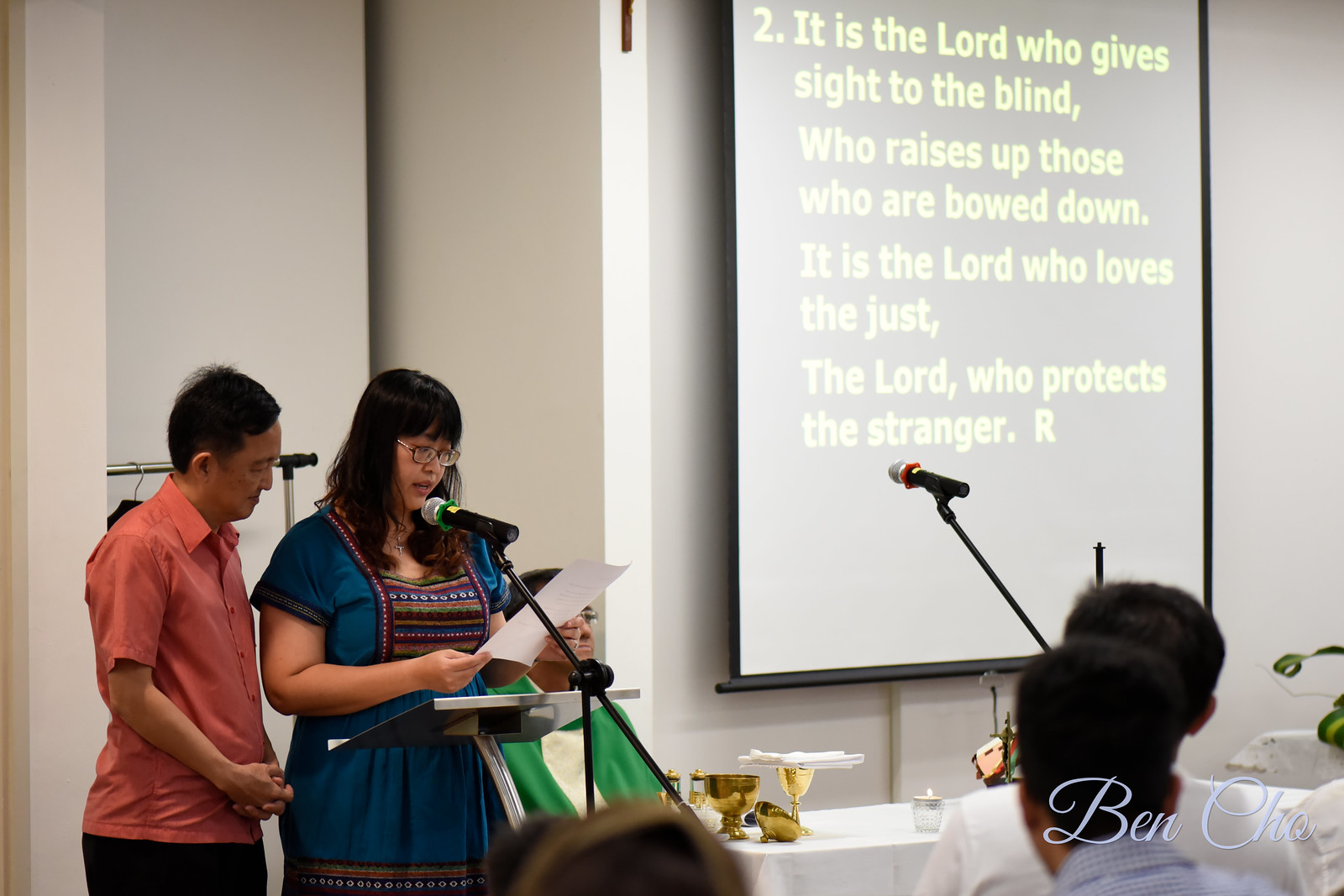The indoor image captures a detailed scene featuring two people speaking at a podium with a microphone. On the right stands a woman of possibly Asian or Hispanic descent, wearing glasses and a teal blue dress adorned with multicolored Native American-style detailing. She has long dark brown hair with bangs and light brown skin. She holds a white piece of paper and is reading from it, her mouth slightly open. To her left is an older gentleman with short black hair and light brown skin, clad in a short-sleeved salmon-colored button-up shirt. He stands with his hands clasped, slightly bent forward to look at the paper the woman is holding. Both individuals appear to have Asian or Hispanic features.

Surrounding them is a meeting hall setup with various attendees, some with short black hair, visible in the bottom right corner of the image. Behind the speakers, a large white screen displays a projected text in white lettering. The legible part of the text reads, "It is the Lord who gives sight to the blind, who raises up those who are bowed down. It is the Lord who loves the just, the Lord who protects the stranger." The screen also partially shows the letter "R" and a signature in light bluish-purple, reading "Ben Cho," presumably the photographer’s credit. A table covered with a white tablecloth and other items is visible along with another microphone in front. This photograph is in landscape orientation and captures a representational realism style.